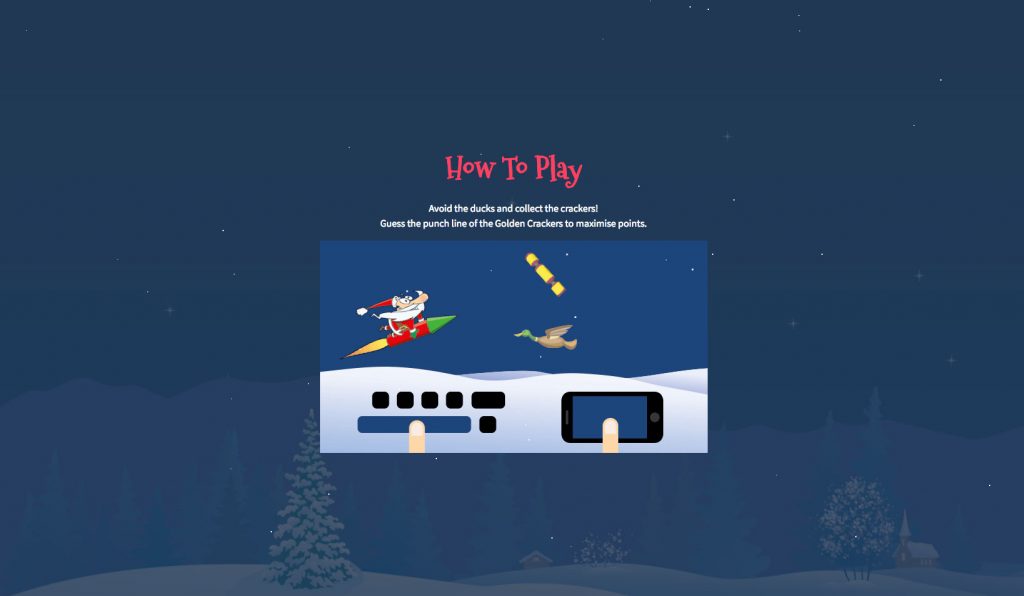In this image, the central focus is on a game screen set against a dark blue background, evoking a nocturnal, winter scene. The bottom portion of the scene features the rolling surfaces of a few snow-covered hills adorned with two barren winter trees. In the middle of the image, text in pink reads "How to Play," followed by two lines of white instructional text detailing the gameplay mechanics. 

Directly below the instructional text, there is a square section displaying a snippet of the actual gameplay. Visible within this square, a rocket ship piloted by Santa Claus, recognizably wearing his iconic Santa hat, soars through the scene. To the right of the rocket ship, a white dove flies alongside, and a diagonal arrangement of golden dots and a block adds visual interest to the sky above Santa. 

At the bottom of this section, the snowy ground is visually punctuated by an assortment of dark geometric shapes: four black squares, one black rectangle, a sizable dark blue rectangle, and an additional misaligned black square. 

In the lower right corner of the image, there is a depiction of a cell phone display, emphasizing the control scheme. Players are instructed to place one finger on the spacebar and one finger on the screen, suggesting how to interact with the game. This setup rounds out the details and instructions presented within this informative, visually structured image.